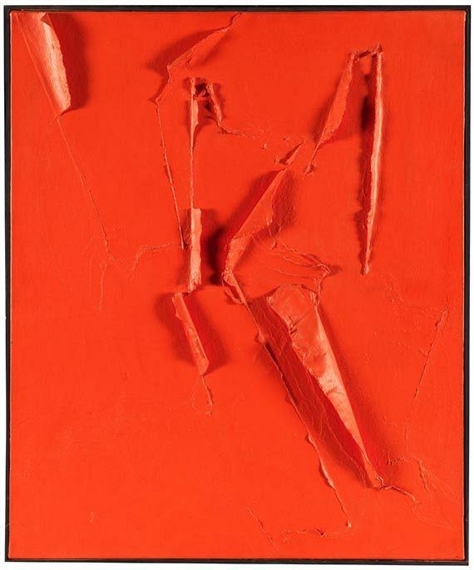This piece of abstract art, called "Tulle Rouge Flemme," features a predominantly tomato-red background with a reddish-orange hue. The painting is rich in texture, ranging from raised triangular areas to various smudges and lighter gradients of red, with shadows adding depth. Towards the upper left-hand corner, there is a small, approximately two-inch section where the paint appears chipped, possibly revealing an underlayer of wallpaper. Central to the artwork are several three-dimensional elements that protrude from the flat plane, resembling papier-mâché or glued-on figures. Notably, in the lower right-hand corner, a carrot-shaped form is one of the most prominent raised features. Adjacent to it is a thin, white streak resembling a pencil, flanked by shapes reminiscent of leaves and flags on skinny flagpoles. These flag-like figures also appear in the upper left-hand corner, sticking out from the surface. Fine lines and subtle cuts give the impression of brush strokes and add to the layered complexity of the piece. This visually engaging work combines geometric shapes, organic forms, and textural contrasts into a cohesive yet enigmatic composition.